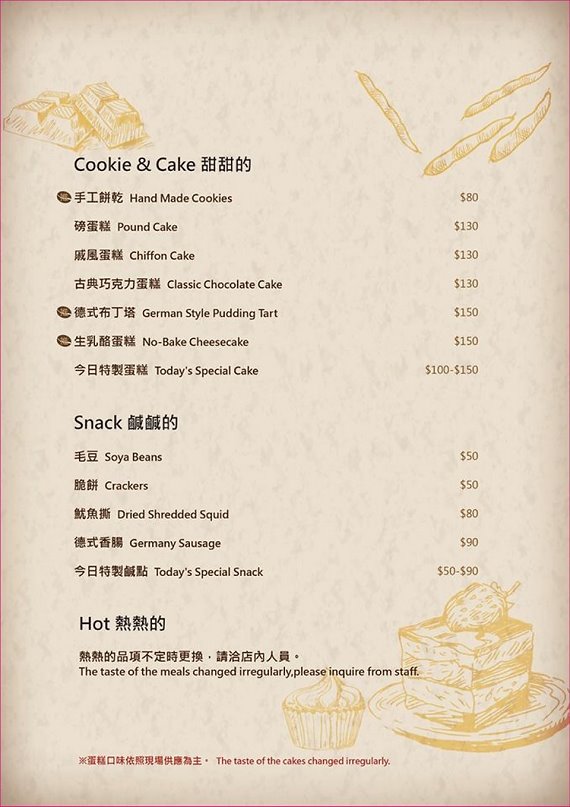The image is a detailed, slightly worn beige menu, likely from a small cafe, presented in both English and Chinese. The menu is organized into three distinct sections: "Cookie and Cake," "Snack," and "Hot." It features black text, with a cream-colored background and stylized illustrations of a chocolate bar, vanilla beans, a cake with a strawberry on top, and a cupcake. The "Cookie and Cake" section lists items such as handmade cookies ($80), pound cake, chiffon cake, and classic chocolate cake (each $130), German style pudding tart and no bake cheesecake (each $150), and today's special cake ($100 to $150). The "Snack" section includes soya beans and crackers (each $50), dried shredded squid ($80), Germany sausage ($90), and today's special snack ($50 to $90). The "Hot" section advises that the taste of the meals changes irregularly, instructing customers to inquire with the staff. The menu has consistent pricing details for each item and occasional notes in red, emphasizing the variability of certain dishes.